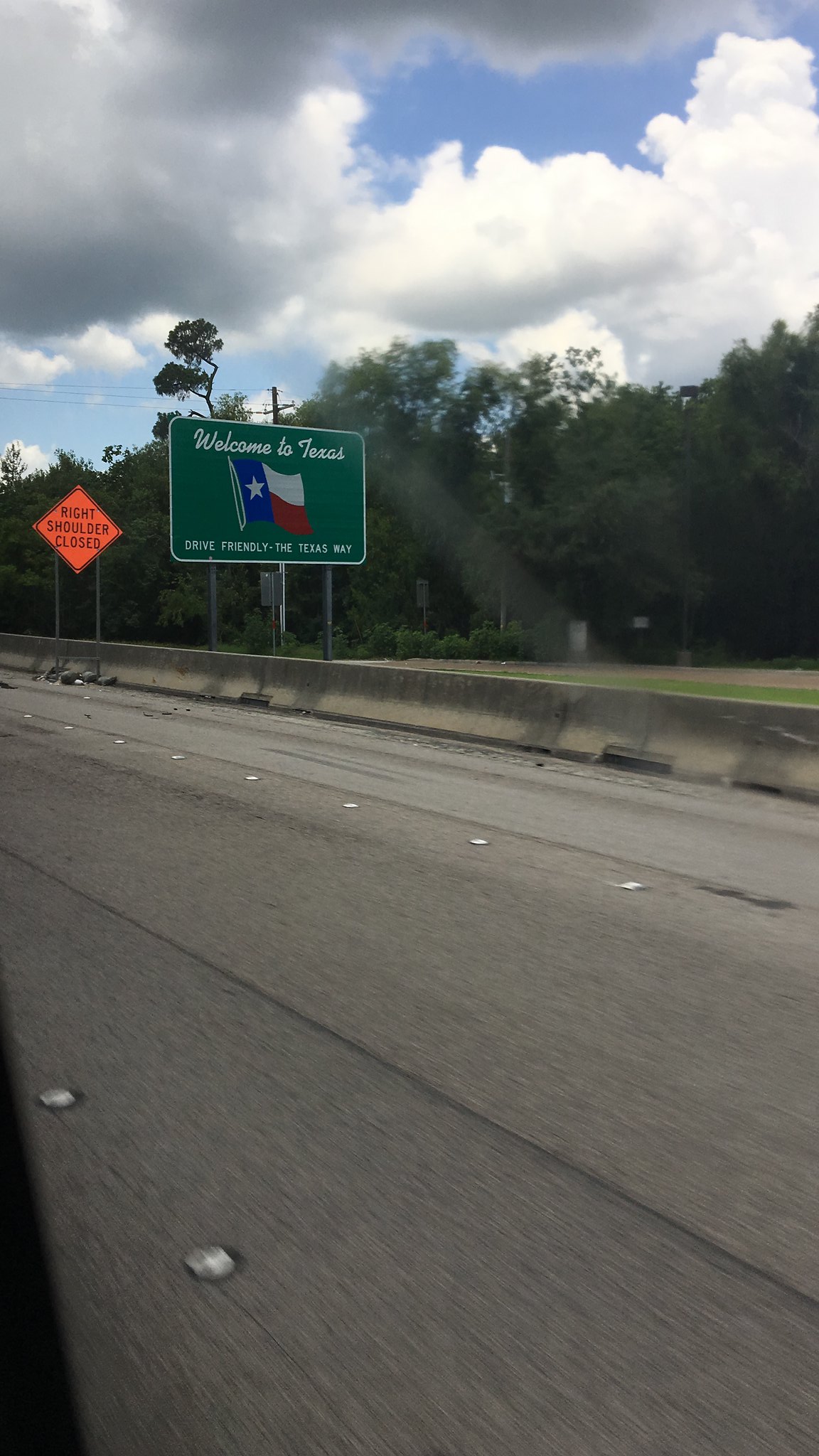A scenic view captured from the right-hand side window of a moving vehicle, showcasing the transition into the state of Texas. The image is taken through glass, though the exact size of the window and the type of vehicle remains unspecified. It reveals a stretch of a three-lane freeway, with two lanes visible on the right. Prominently displayed is an orange triangular sign indicating "Right Shoulder Closed," juxtaposed with a larger green sign welcoming travelers with "Welcome to Texas" and the Texas flag, alongside the slogan "Drive Friendly - The Texas Way." In the background, the horizon is dotted with trees and patches of grass, bathed in the soft light of a daytime baby blue sky adorned with scattered clouds. The setting suggests a peaceful journey as the photographer captures a moment of travel through the Lone Star State.